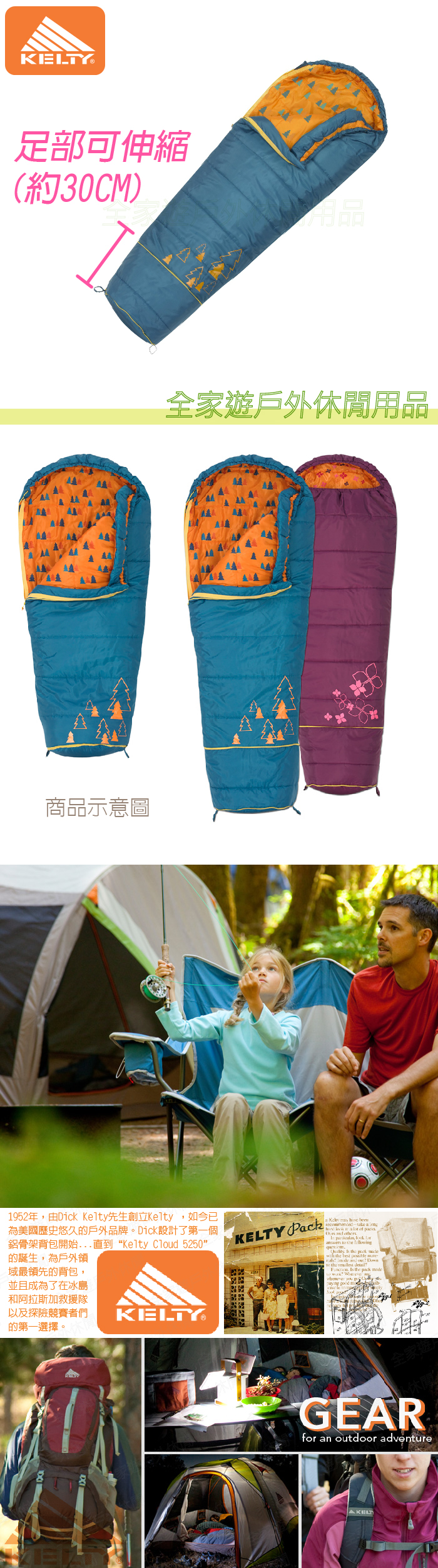This advertisement, featuring what appears to be a sleeping bag, is presented in a long and narrow format and written in an Asian language, recognizable by its symbolic script. The ad is divided into four main images sequentially arranged down the page:

1. At the top, a blue sleeping bag with an orange interior is displayed. The bag is unzipped to reveal its vibrant inside, with pink text to its left indicating the item's length as 30 centimeters.

2. The second image shows three sleeping bags: two are pink with orange interiors. Alongside these, a man and a young child are seated in camping chairs, with a tent and fishing rods visible in the background, suggesting a family camping scene.

3. Below this, the ad prominently displays the word "GEER" and the brand name "KELTY."

4. The final section includes small photographs of people engaged in various outdoor activities like hiking, further promoting the adventurous spirit associated with the product.

Overall, the advertisement effectively blends detailed product imagery with lifestyle scenarios to appeal to potential buyers.